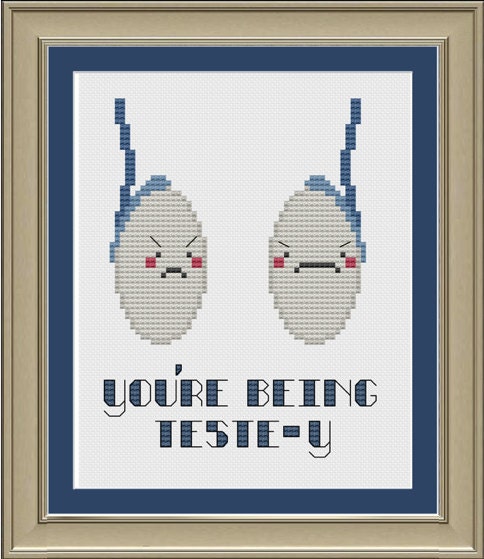This detailed image showcases a meticulously crafted cross-stitch framed in an ornate silvery-bronze frame. The stitched artwork is bordered by a vivid blue outline and sits against a clean white backdrop. At the center of the composition are two egg-shaped figures, each created with gray cross-stitches and adorned with subtle blue accents extending from their tops. These figures display distinct faces with frowny, grouchy expressions—one eggs' face is further detailed with red and black accents and blushing cherry cheeks. Above the stern faces, bluish rectangles rise, adding a distinctive visual element. The figures appear to interact with each other, one gazing directly outward while the other looks to the side. Below this intriguing scene, the text "You're being testy" is stitched in large, fancy, squarish letters, subtly hinting at a playful critique, making it an endearing piece for those with a well-meaning attitude.